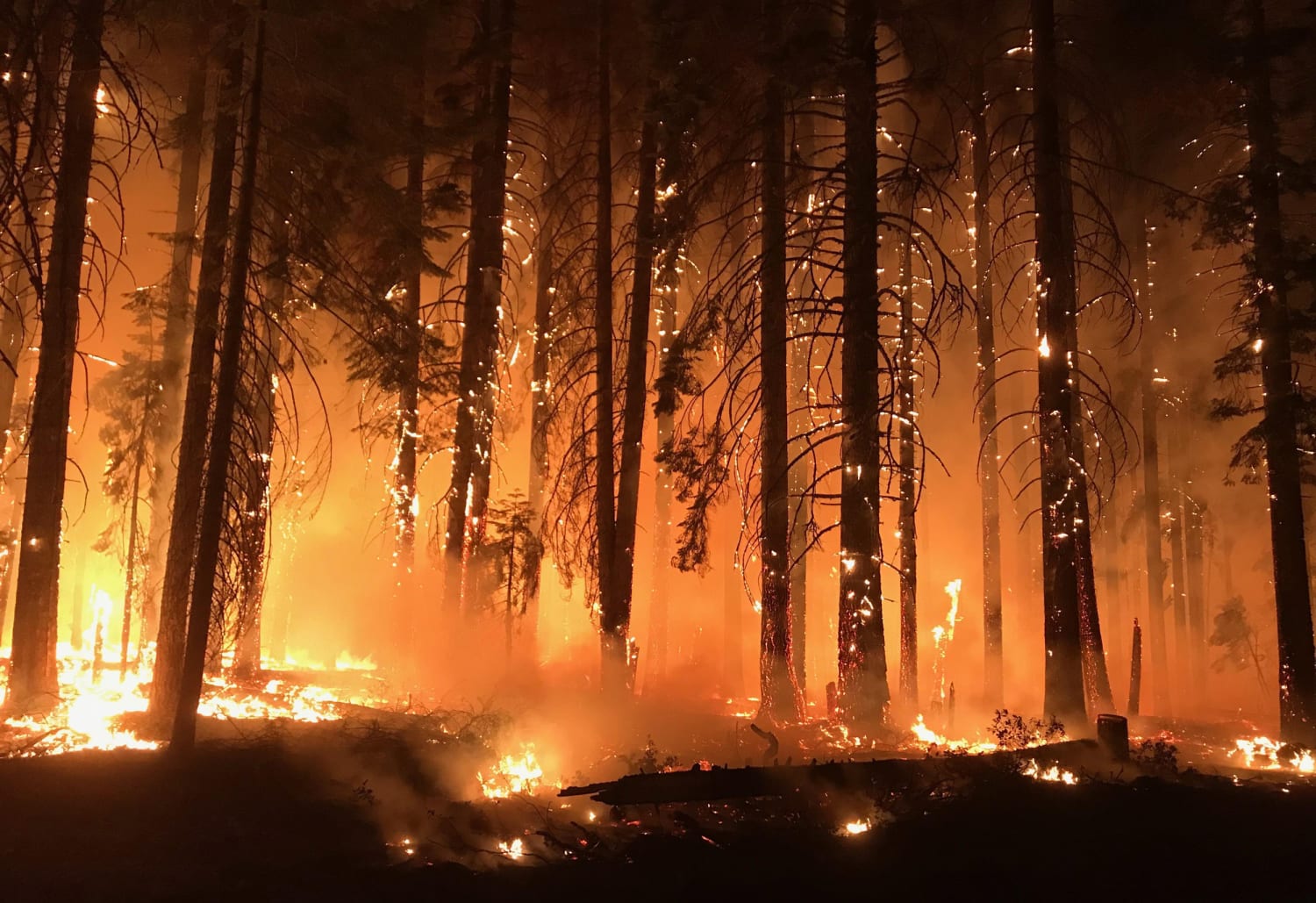This horizontal rectangular image vividly captures the intense destruction of a forest fire amidst a dark and smoky background. In the foreground, spots of flames scorch the ground, while an orange-y light further illuminates the forest as the fire advances. The tall, skinny trees stand lifeless with drooping branches, many of which have been stripped of leaves and are engulfed in flames. The bark of the trees glows intensely, with the fire seemingly cascading down the trunks. On the left side of the image, the flames burn fiercely with a bright white color, signifying greater intensity that spreads towards the right side and forward. The scene is engulfed in a thick, grayish haze of smoke, adding to the chaotic atmosphere of destruction. Fallen branches litter the ground, further accentuating the devastation. The overall impression is one of overwhelming chaos, with fire consuming everything in its path and reducing the once-vibrant forest to a smoldering ruin.